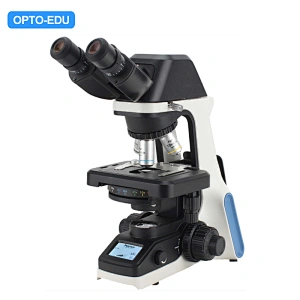This image features a sophisticated educational microscope labeled with the brand "Opto-EDU" displayed prominently in a blue banner at the top of the photo. The microscope is designed with two black binocular eyepieces for stereoscopic viewing. It has a robust, white structural arm complemented by black components and a distinctive blue accent near its base. The device includes three adjustable objective lenses or magnification scopes, each marked by colored stripes for easy identification. Additionally, the microscope has a unique small rectangular screen positioned at the bottom, likely used for displaying data or images captured through the lenses. The stage, where slides are placed, is black, with silver metal clips to secure the slides in position. Black adjustment knobs are located on the side, allowing precise control of the focus and magnification. The overall photograph appears to be taken from a side-diagonal angle, emphasizing the elegant and functional design of the microscope.